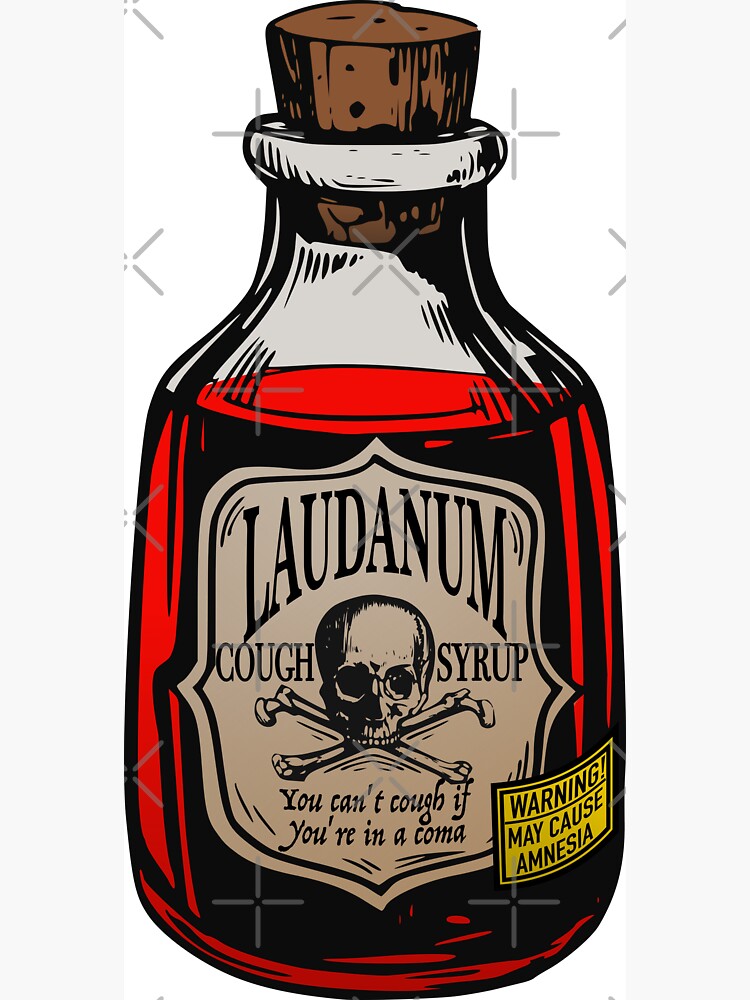The image presents a whimsical and illustrative design of a fictional product called "Laudam Cough Syrup." The bottle, which is depicted in a black color with a deep red liquid inside, is topped with a slightly uneven brown cork stopper. The graphic design features a gray background with light gray sparkle shapes, providing an artsy and less realistic look. Prominently displayed on the front of the bottle is a label that reads, "Laudam Cough Syrup," accompanied by a skull and crossbones symbol. Beneath this, the text warns, "You can't cough if you're in a coma," emphasizing the dark humor. To the right-hand side of the bottle is a bright yellow rectangular warning label stating, "Warning: may cause amnesia," in all capital letters. The bottle appears about 80% full and the overall aesthetic suggests a cartoony, likely fabricated product intended for a humorous effect.